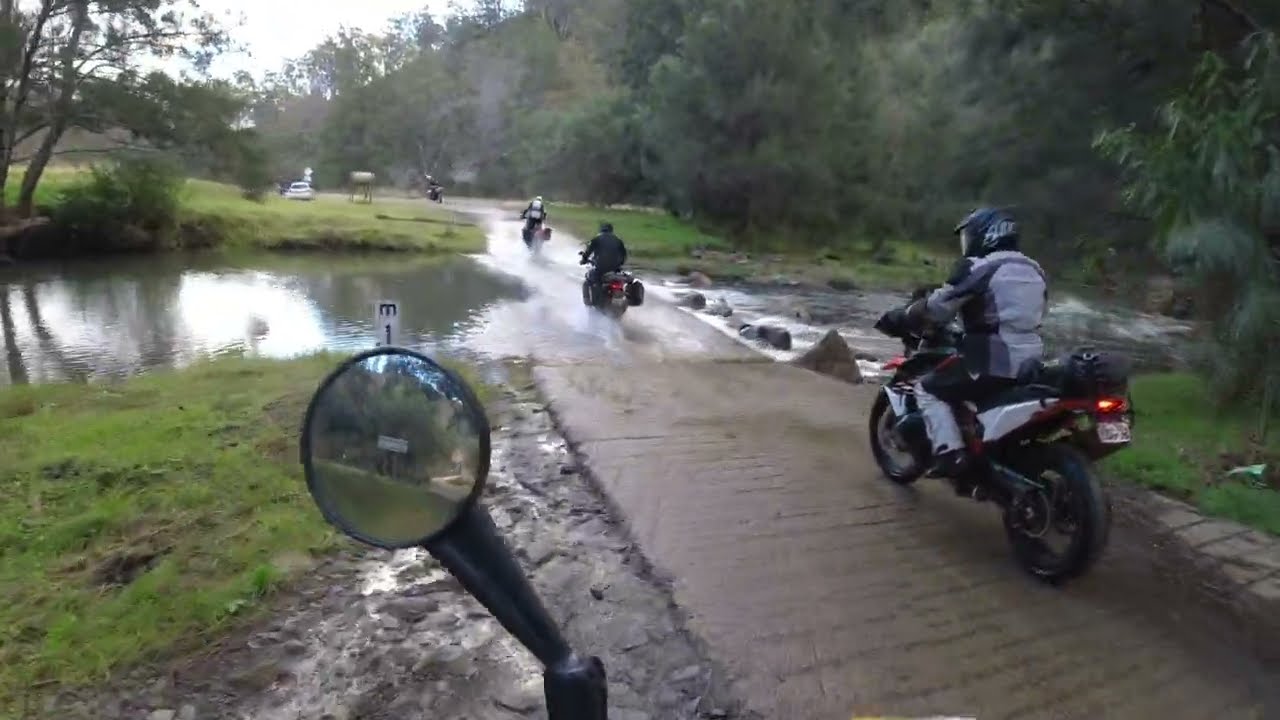In this color photograph, captured from a GoPro camera mounted on a motorcyclist's handlebars, we see a dynamic scene from the rider's perspective. On the front left, the circular rearview mirror on a black handle is prominently visible. The scene is set on a dirt path that appears to rotate 45 degrees counterclockwise, extending from right to top-left, transitioning from a wood-brown plank pathway to a stone-gray road. Multiple motorcyclists are navigating this path. Closest to the camera is a rider on a red and white Kawasaki-style motorcycle, clad in a black helmet and a white, gray, and black full bodysuit. Ahead, another rider in a similar jumpsuit and dark helmet can be seen riding a white scooter further along the path. The path crosses a river, where two motorcyclists are captured splashing through the water, while another is seen emerging from the river on the other side. The background features a verdant landscape with green fields and bushes to the right, a scattering of trees at the river's edge, and hills faintly visible in the far distance. The scene exudes a sense of adventure and motion, with the motorcyclists braving the rugged terrain in a scenic countryside, beautifully presented in a freeze-frame style.